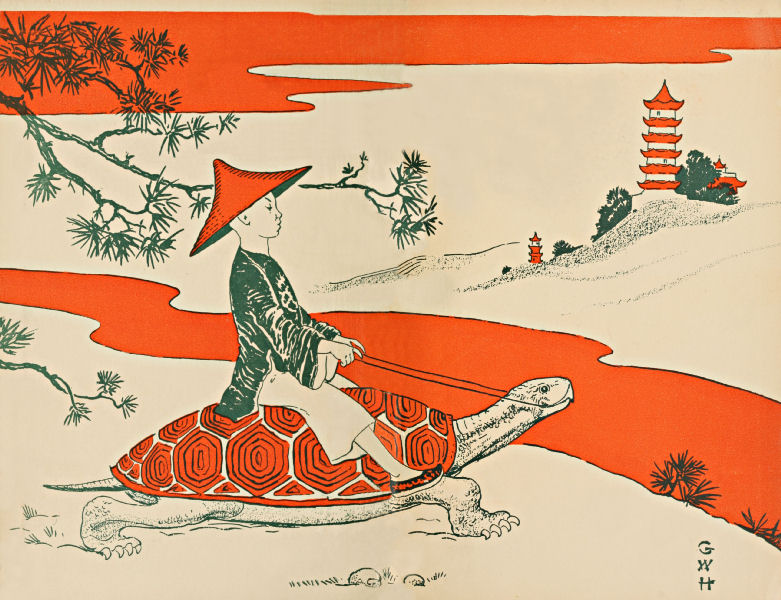The illustration appears to be an oriental-style graphic filled with vibrant hues of orange, green, and beige. A young man, possibly Asian, is the central figure, wearing a straw hat reminiscent of Raiden from Mortal Kombat and a green jacket paired with beige or white pants. He rides an imposing orange-shelled tortoise, guiding it with a thin harness attached to its mouth. The tortoise is making its way towards an orange-hued river, adding to the fantastical ambiance of the scene. 

In the background, there is a traditional Japanese-style temple with tiered roofs, depicted in orange and beige tones, standing tall amidst green trees and branches extending into the frame. The sky above features rich orange clouds, creating a surreal sunset-like effect. The details – such as the string reins held by the man, the gentle progression of the tortoise, and the intricate background elements – come together to create a vivid, storybook-like quality to the image. The letters "GWH" can be seen on the side, possibly indicating a signature or title. Overall, the captivating scene highlights a journey through a mystical landscape, blending traditional motifs with imaginative elements.